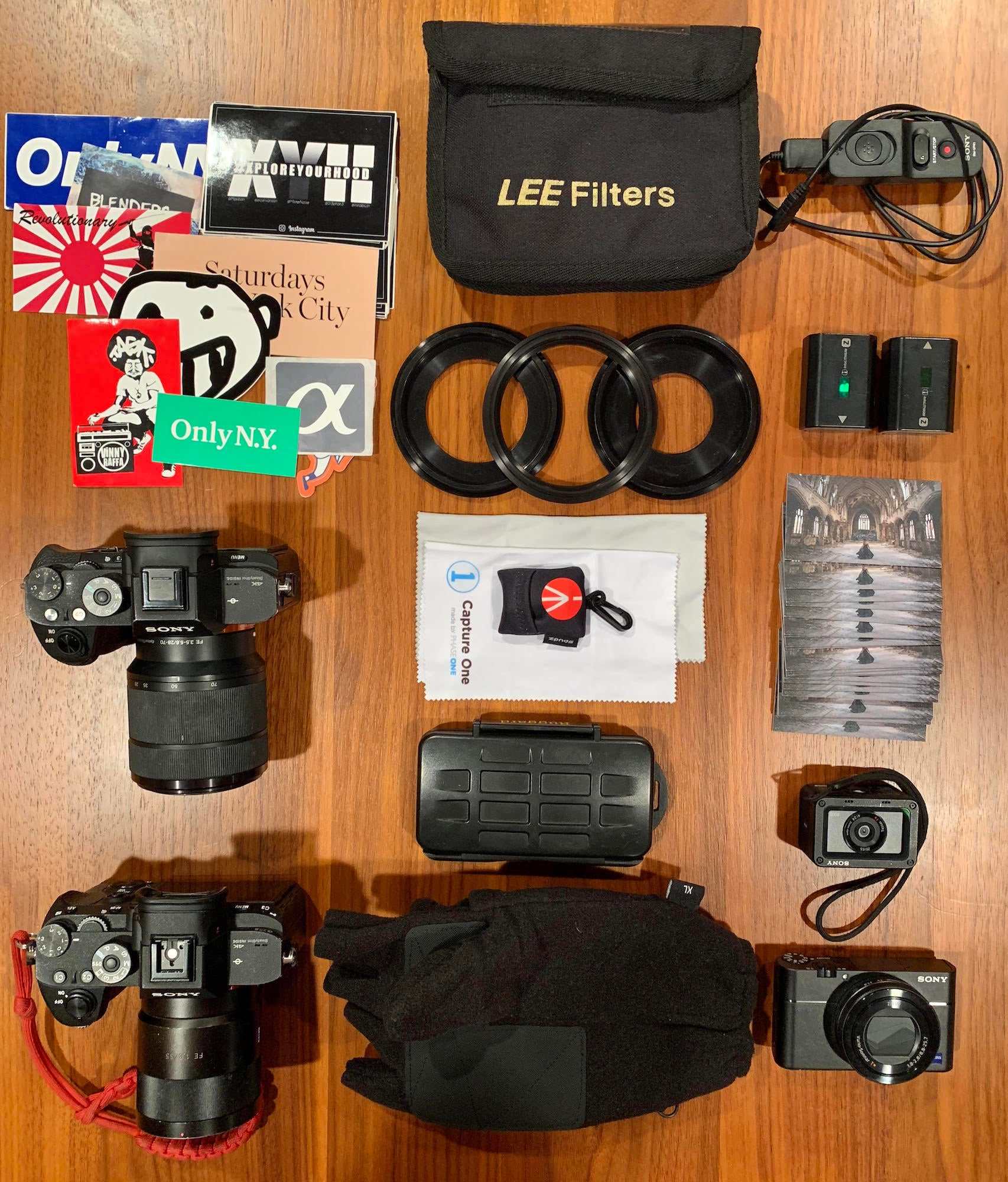A meticulously organized array of camera equipment is spread across a wooden table, reminiscent of vinyl wood commonly found in conference rooms. On the left side, there is a sturdy case designed to carry camera lenses. Nearby, a cable snakes its way across the table alongside several small packs, possibly battery packs. Just below these items lies a neat stack of identical photographs. In the upper left corner are a few black rings, likely lens caps or filter rings. Scattered around them is a colorful assortment of cards in hues of blue, black, red, white, green, and gray. To the right, two Sony cameras with long lenses rest prominently, testament to their professional quality. In the bottom right corner is another camera, and just above it, a smaller camera is positioned. Nestled between these is a black case, possibly housing additional equipment.